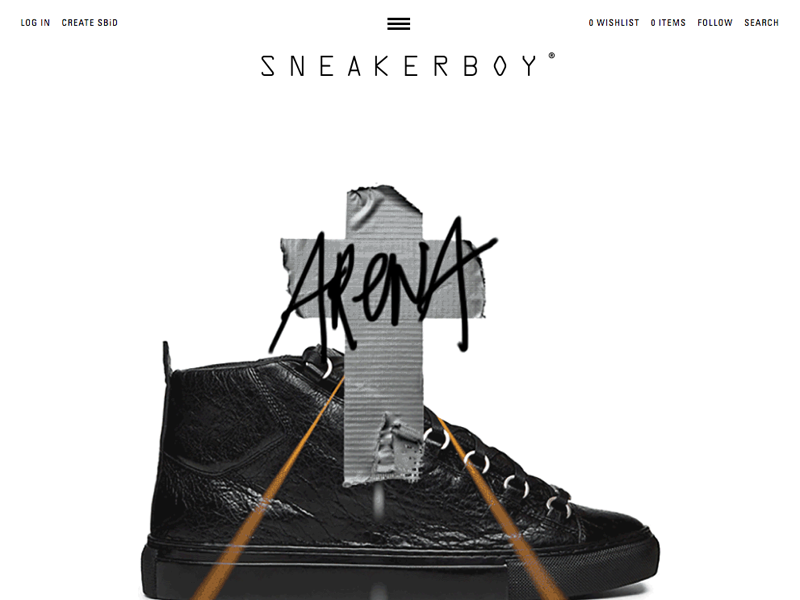The image appears to be a screenshot of a website with a white background, prominently displaying the name "Sneaker Boy" in all capital letters using a retro computery font, with a registered trademark symbol on the upper right. At the top of the screen, from left to right, there are navigation elements: "LOGIN" and "CREATE SBID" in capital letters, followed by a hamburger menu icon in the center, and "ZERO WISHLIST," "ZERO ITEMS," "FOLLOW," and "SEARCH" also in capital letters to the right. 

Dominating the central part of the image is a graphic of a black, low-top sneaker with a textured leather exterior and silver ring loops for the laces. Overlaid on the sneaker is a cross made of two pieces of silver duct tape, with the word "ARENA" written across the tape in a sharpie-like or graffiti-style font. Two yellow-orange beams emanate from the duct tape cross on either side, adding a striking visual element. The sneaker faces to the right and is set against the overall clean, white design of the webpage.